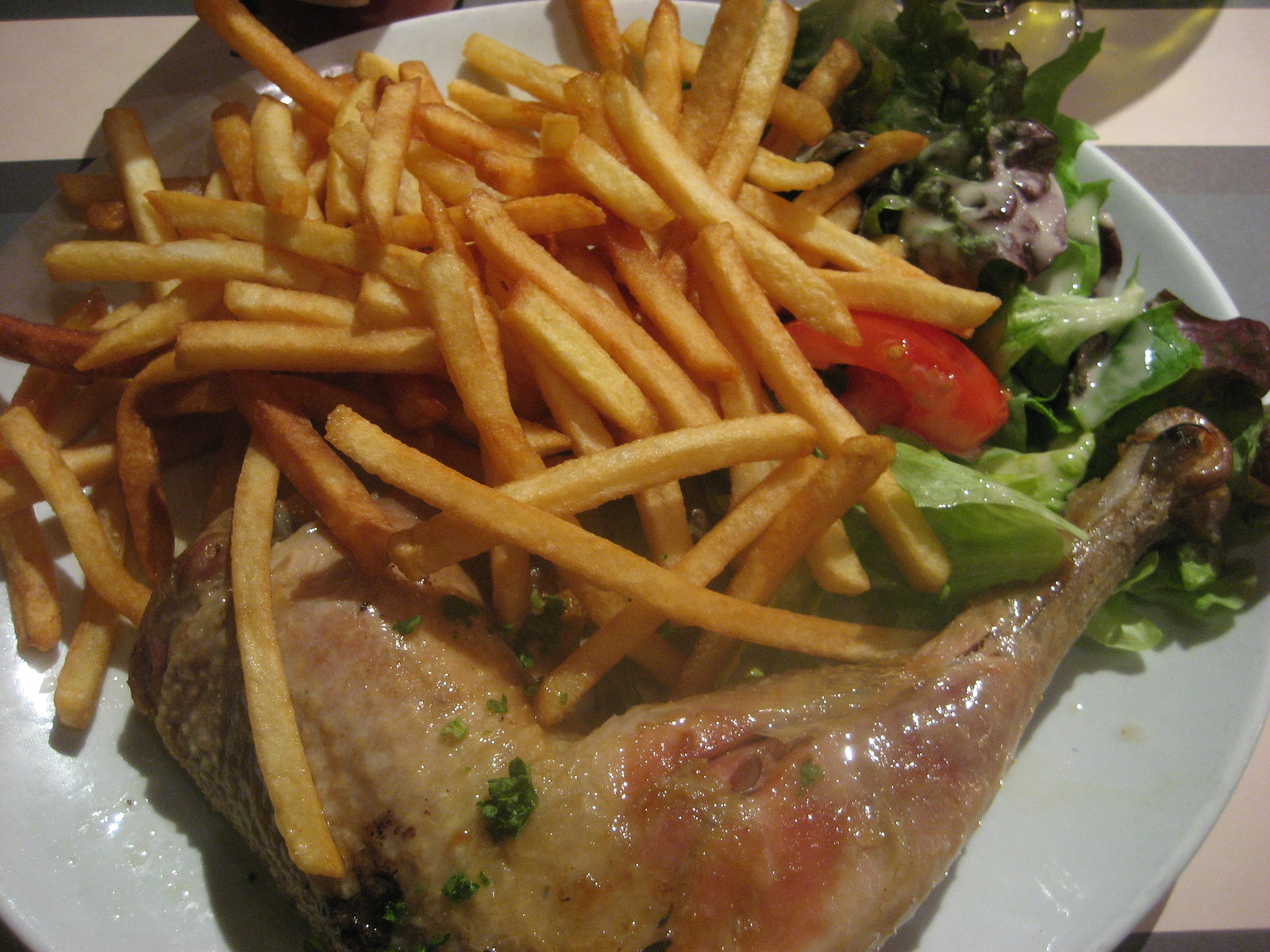This photograph showcases a white, round porcelain plate against a background that transitions from pinkish roan to gray. The focal point of the plate is a long chicken leg and thigh, appearing baked with possible herb garnishes. The chicken, with its slightly bumpy skin, sits towards the bottom of the plate. Centrally positioned and extending to the left are a generous serving of straight-cut, golden-brown french fries. On the upper right side of the plate lies a vibrant side salad consisting of mixed green and purple lettuce, a slice of red tomato, and a drizzle of white dressing, possibly ranch. The overall scene features subtle shadows at the top, creating a sense of depth in the image.